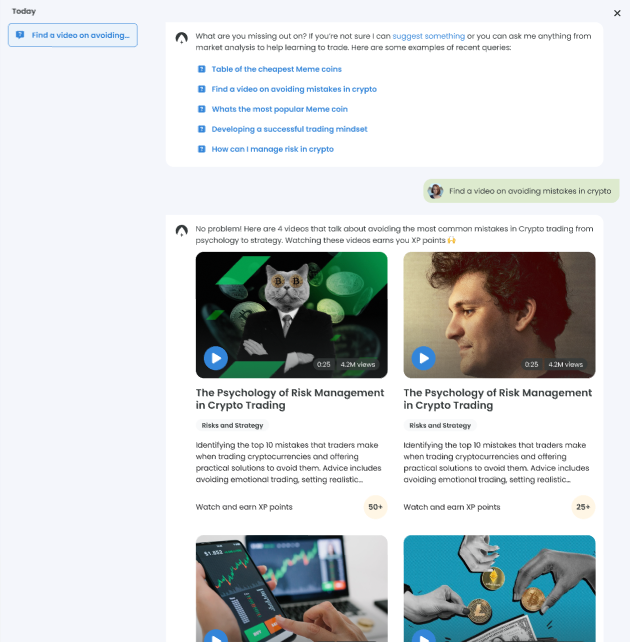The image features a split background, with the left side being a very light blue and the right side transitioning to black. At the top, "Today" is written in black text against the background. Below that, a blue rectangle with a darker blue outline contains the text "Find a video on avoiding…" indicated by an ellipsis.

Adjacent to this on the right, a white rectangle bears the prompt, "What are you missing out on?" in black text at the top. Below, the text continues in black stating, "If you're not sure I can suggest something," followed by another portion in black, "or you can ask me anything from market analysis to help learning to trade. Here are some examples of recent queries." The segment transitions into a blue background featuring a white question mark, along with a list of bullet points in blue text:

1. Table of the cheapest meme coins.
2. Find a video on avoiding mistakes in crypto.
3. What's the most popular meme coin?
4. Developing a successful trading mindset.
5. How can I manage risk in crypto?

Below this section, the background turns gray, and a green rectangle houses the black text, "Find a video on avoiding mistakes in crypto."

Further down, another white background appears, containing the statement: "No problem. Here are four videos that talk about avoiding the most common mistakes in crypto trading from psychology to strategy. Watch these videos to earn XP points." The listed videos include:

1. The psychology of risk management in crypto trading.
2. The psychology of risk mismanagement in crypto trading.
3. (Titles for the remaining two videos are not visible.)

This detailed layout provides a comprehensive guide on finding resources and common questions related to crypto trading mistakes and strategies.